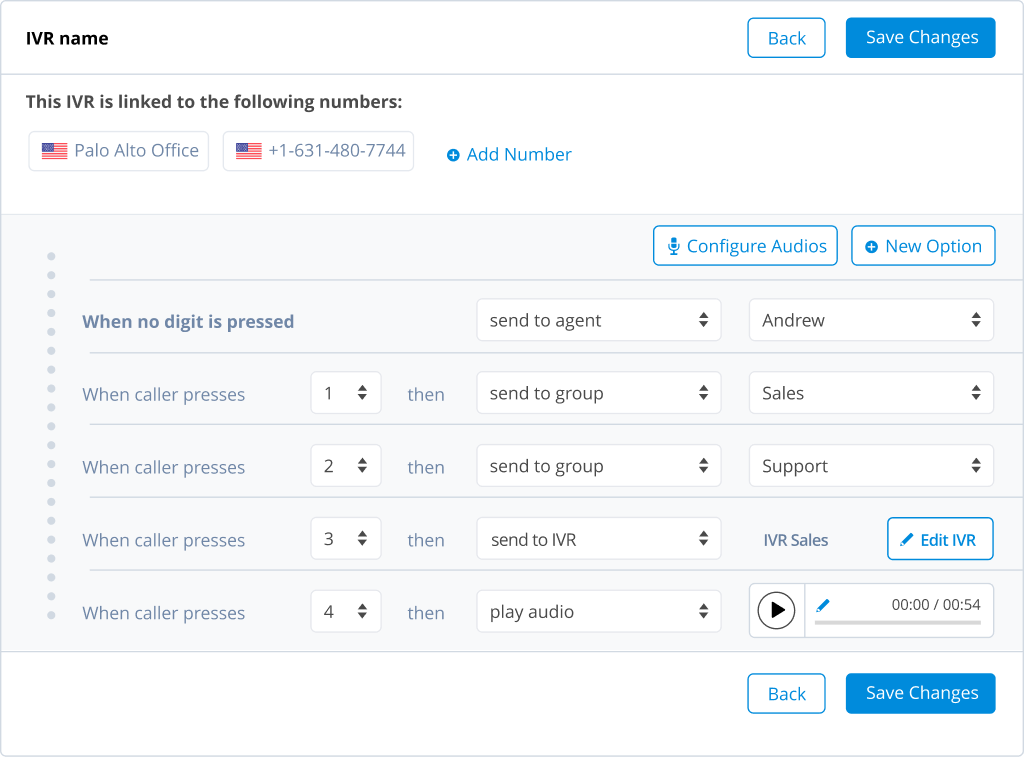**Image Description: Interactive Voice Response (IVR) Configuration Form**

The image features a landscape-oriented user interface for configuring an Interactive Voice Response (IVR) system. 

1. **Layout & Buttons**:
   - At the **upper left corner**, the header is labeled "IVR Name".
   - At the **upper right corner**, there are two buttons: a "Clear Back" button in a neat, simple design, and a "Save Changes" button highlighted in blue.

2. **Background**: The overall background is a clean, white canvas that makes the content stand out distinctly.

3. **Sections**: 
   - **Gray Stripe**: A horizontal gray stripe separates the header from the main content sections below.
   - **Linked Numbers Section**:
     - This section's header states, "This IVR is linked to the following numbers".
     - It includes two buttons:
         - **Left button**, displaying an American flag icon and the text "Palo Alto Office".
         - **Right button**, also with an American flag icon, followed by a specific phone number.
     - A blue hyperlink labeled "Add Phone Number" is available beneath these buttons, allowing new numbers to be linked.

4. **Configuration Section**: 
   - This area has a slightly darker white-gray background.
   - **Right Side**:
      - Two main buttons: "Configure Audios" and "New Option".
   - **Routing Instructions**: 
      - Below these buttons, there are various routing instructions:
         - "When no digit is pressed, send to Agent Andrew".
         - "When caller presses 1, send to Group Sales".
         - "When caller presses 2, send to Group Support".
         - "When caller presses 3, send to IVR Sales", with an option to edit this IVR.
         - "When caller presses 4, play audio", with an interface to listen to the selected audio for a duration of 54 seconds.

5. **Bottom Section**: 
   - Similar to the top, the bottom right corner includes a "Clear Back" button and a blue "Save Changes" button.

The overall design of the form is user-friendly, with clear sections and buttons to streamline the configuration process of the IVR system.